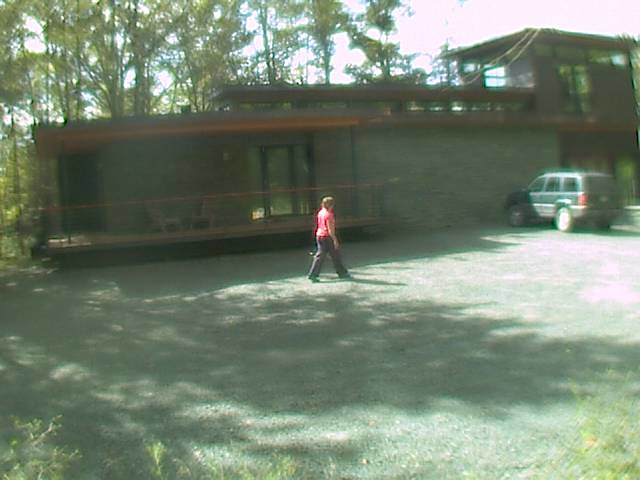The photograph captures a detailed outdoor scene featuring a narrow and long building, which appears to be set in a wooded area with several large trees in the background. The building is primarily single-storey with a flat roof, except for a cuboid-shaped two-storey section on the right that has large glass windows. The exterior of the building features gray brick or siding, accompanied by a large veranda with a glass entrance door. 

In the foreground, there's a gravel parking lot interspersed with patches of grass, twigs, and leaves. A woman with short hair and light skin is walking from left to right across the parking lot. She is wearing a pink shirt and dark trousers. The woman is heading towards a green SUV parked in front of the building. The photo is taken during the day, evident from the bright sky and the shadows cast on the gravel. The vibrant greenery of the trees and the overall composition add a serene yet dynamic feel to the image.